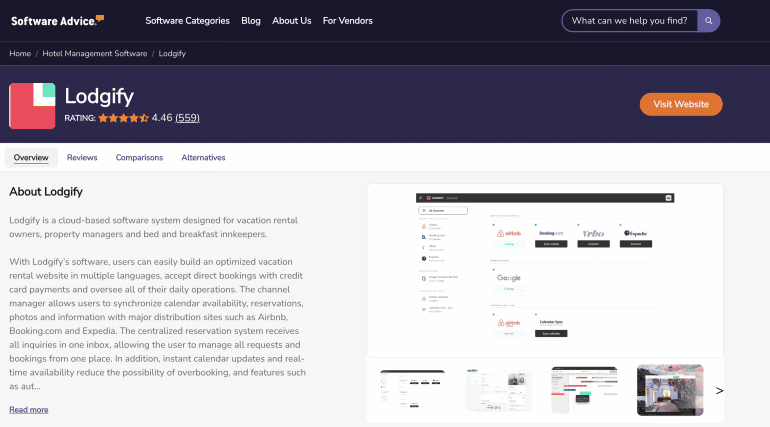Caption: 

The image showcases a web page from Software Advice. In the upper left corner, "Software Advice" is displayed, followed by navigation links to "Software Categories," "Blog," "About Us," "For Vendors," and on the far right, there's a search bar with the prompt "What Can We Help You Find?" set against a black background with white text. 

Below this navbar, on the left side, it lists "Home," followed by a breadcrumb trail to "Hotel Management Software" and "Lodgify." Underneath this trail, in a blue strip, the name "Lodgify" is prominently featured in white text, accompanied by its spelling, "L-O-D-G-I-F-Y," its rating of 4.6 stars based on 559 reviews. On the right side of this blue strip, there's a bright orange "Visit Website" button with white text.

Further down, on a gray background, several tabs are presented, starting from the left: "Overview," "Reviews," "Comparison," and "Alternatives." Below these tabs, there is a detailed section titled "About Lodgify." This section explains that Lodgify is a cloud-based software system aimed at vacation rental owners, property managers, and bed and breakfast innkeepers. It highlights features such as easy website creation and optimization in multiple languages, direct booking capabilities with credit card payments, and comprehensive daily operation management. Additionally, Lodgify offers a channel manager that synchronizes calendar availability, reservations, photos, and information with major distribution sites like Airbnb, Booking.com, and Expedia.